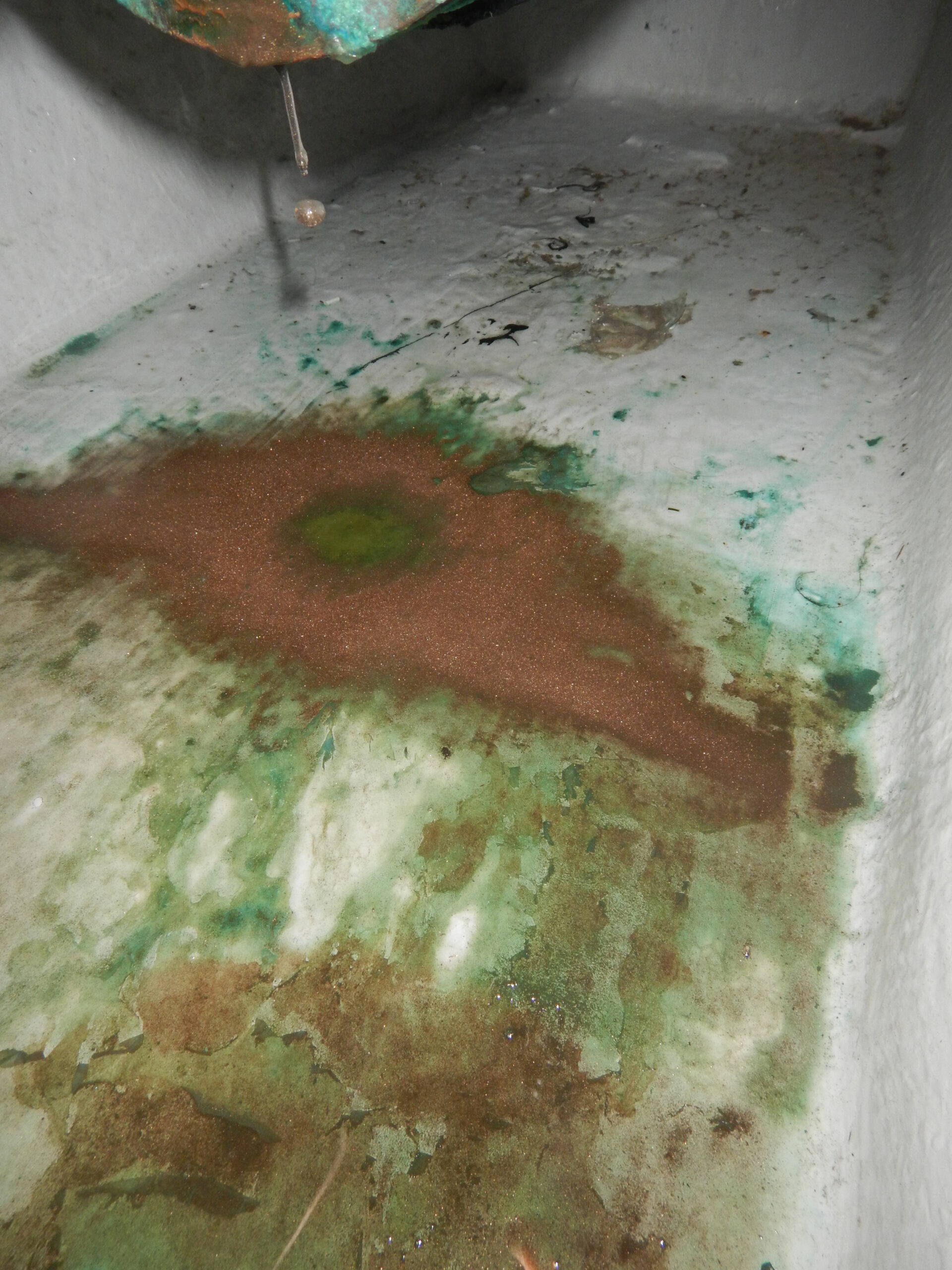This image depicts a long, rectangular chamber, potentially an old concrete container, viewed from one end with the far wall visible a short distance away. The chamber, mostly painted white, shows signs of significant wear, with large rust stains and green streaks running down the walls and floor. At the top of the image, a round, rusty appendage, possibly a pipe, is dripping water, with one drop captured mid-air. The water drop appears to be causing a lighter green circular stain surrounded by a brown area. There are additional green and brown splotches scattered across the floor. Shadows cast by the pipe add to the dim and aged atmosphere, suggesting the chamber's possible use in industrial or mechanical contexts.